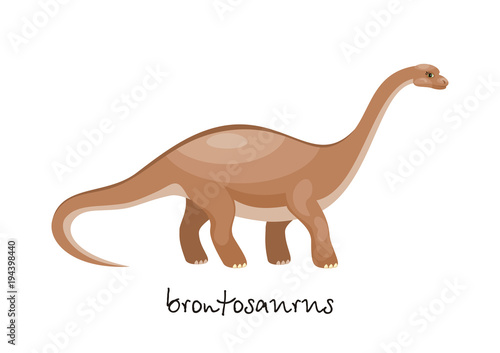The image features a clipart of a light brown brontosaurus, prominently displayed in the right background and facing towards the right with its eyes staring sideways. The dinosaur boasts a characteristic long neck, four thick and wide legs, and a curved back. Its tail, which subtly curls underneath itself (but not under its body), extends toward the left side. The brown coloration of the brontosaurus transitions gradually, with the hues ranging from pale shades on its back to darker browns towards the bottom, and a light brown belly. Across the image, in a cursive black font, the word "Brontosaurus" is inscribed. Additionally, a watermark indicating "Adobe Stock" appears on the left side, along with the reference number 143439A440.